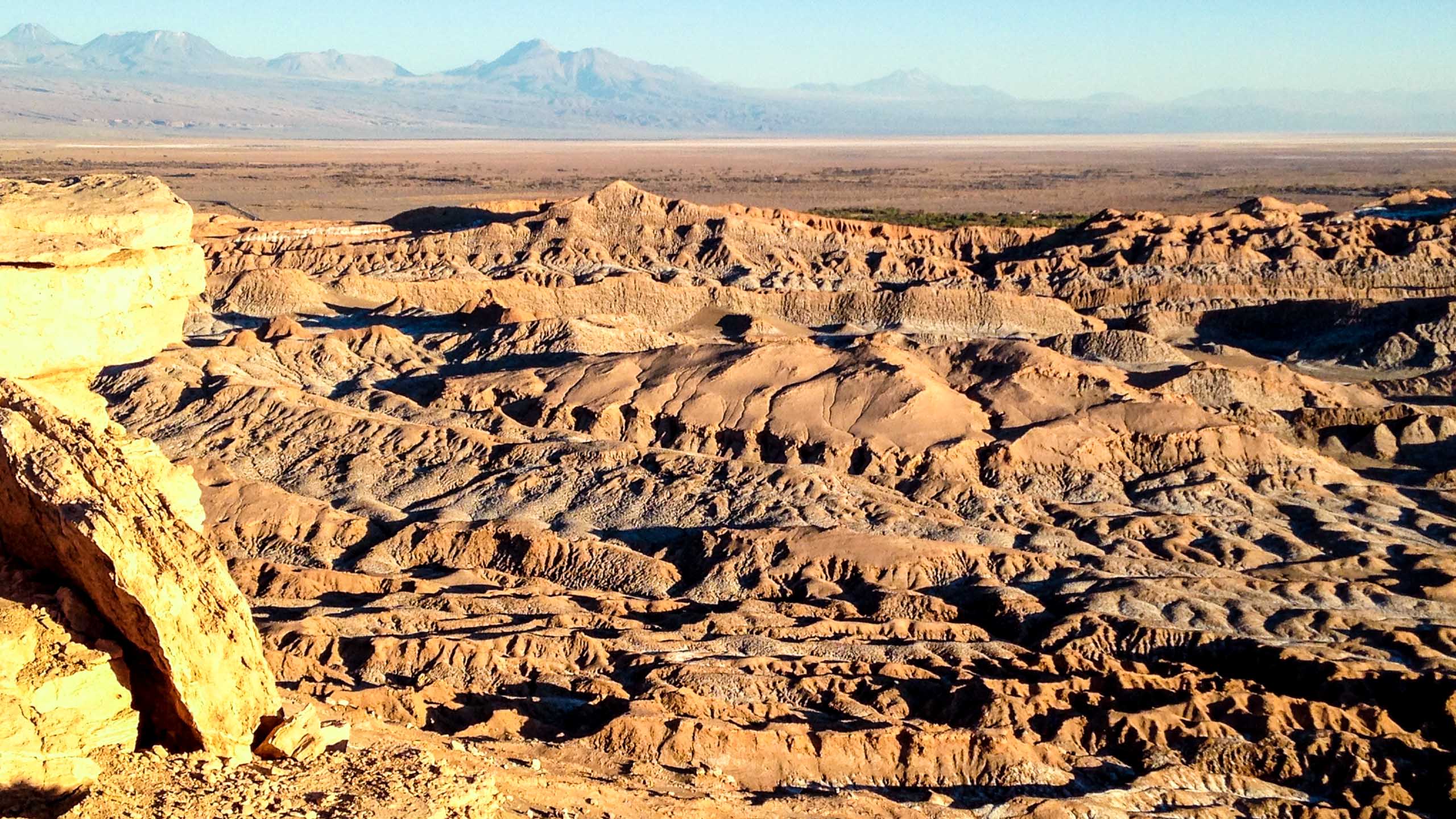The image features an expansive rocky terrain, captured from a higher vantage point. In the foreground to the left, large boulders and yellow rocks stand prominently, part of the elevated area from where the photo is taken. The landscape below is dominated by rugged, weathered hills interspersed with numerous small ravines, hinting at past water flow. Stretching out from these hills is a wide, flat desert plain, eventually meeting a distant, hazy mountain range. The scenery presents a predominantly reddish-brown hue with patches of dry, harsh terrain. The sky above is a clear, vivid blue, enhancing the desolate yet majestic beauty of the scene.